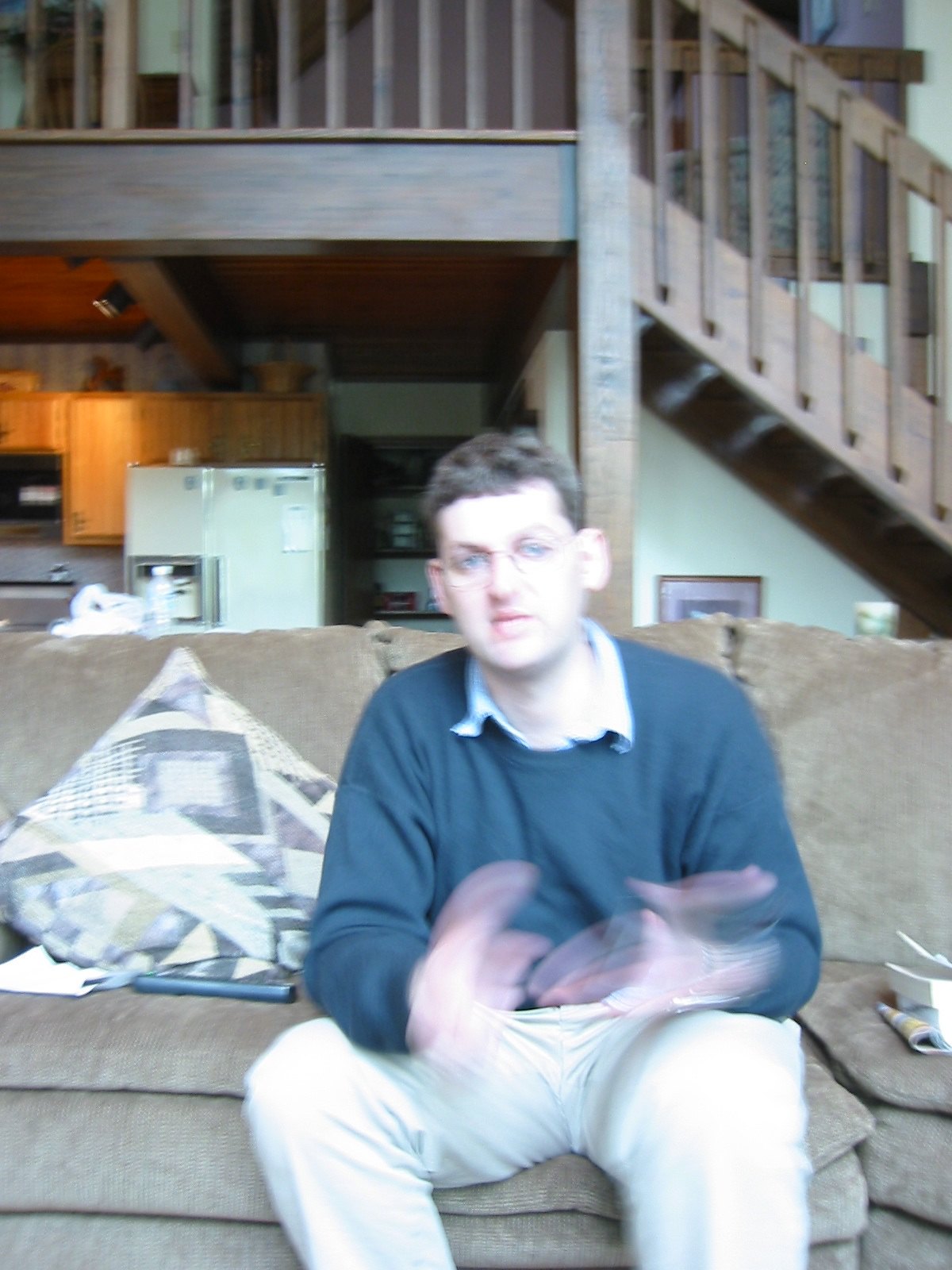A young man in his early 20s is seated on a tan couch located in the living room area of a house. The man has brown hair, wears glasses, and has blue eyes. He is dressed in khaki pants and a blue shirt layered over a collared shirt. His hands appear blurred, suggesting movement, while the rest of the image maintains a general blur, but with identifiable objects and details. To his right on the couch lies a throw pillow, a TV remote, and possibly a book. In the background, the kitchen is visible, featuring an old-fashioned fridge, shelving, and cupboards. Behind him, stairs lead up to a loft area, indicating additional rooms and spaces upstairs.